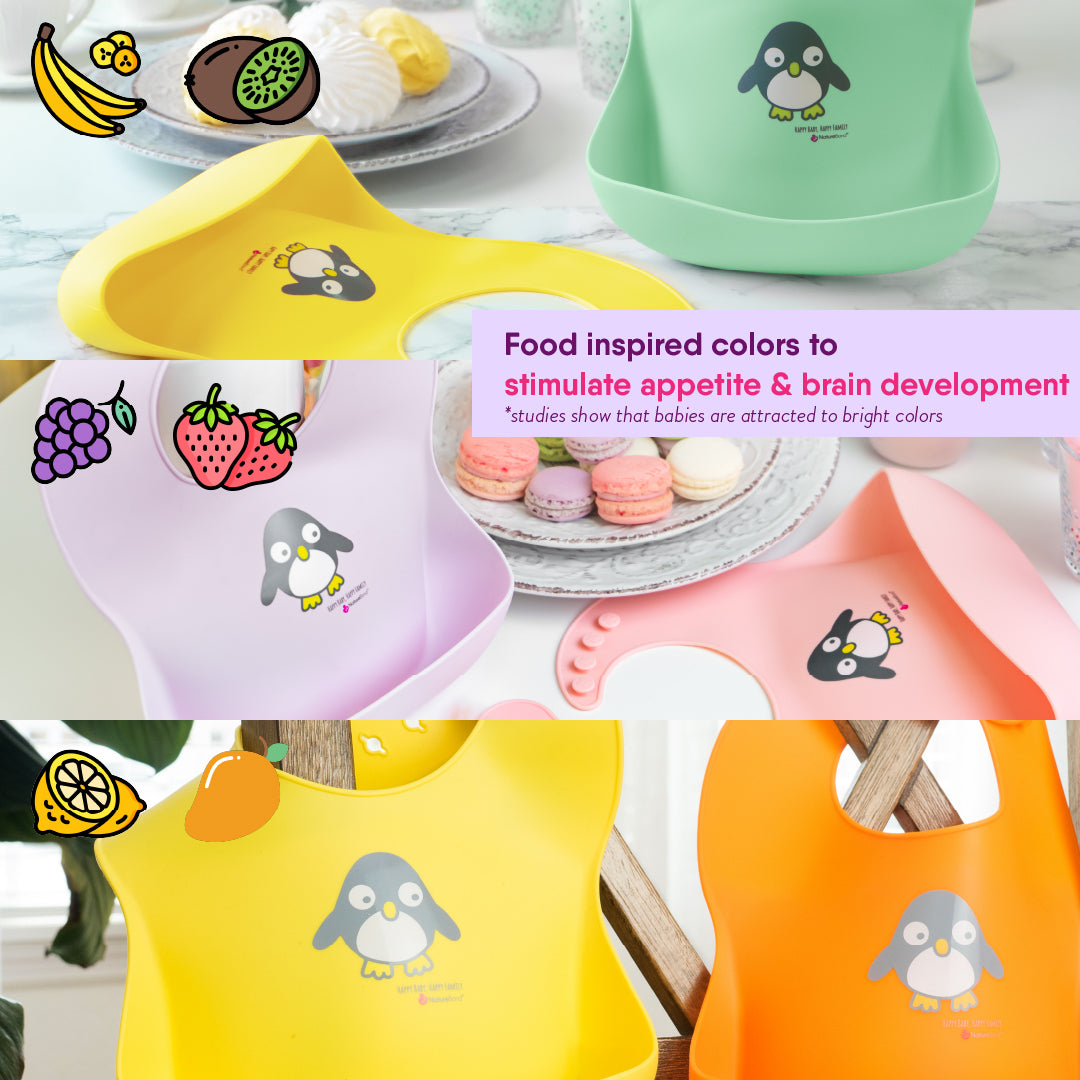This image is a detailed advertisement for silicone baby bibs, presented in a collage format with multiple images. The bibs come in a variety of bright, food-inspired colors, specifically pink, purple, yellow, orange, green, and peach, each designed to stimulate appetite and brain development in babies. Each bib features a pocket at the bottom to catch food, and they are further adorned with a cute penguin cartoon.

The collage layout showcases three sets of bibs from top to bottom. The top row features yellow and light green bibs alongside a small illustration of a banana and a kiwi. The middle row displays light purple and light pink bibs with a grape and a strawberry. The bottom row shows yellow and orange bibs next to a lemon and a carrot. The right side of the image includes a purple rectangle with the text in darker purple and pink highlighting the benefits: "Food-inspired colors stimulate appetite and brain development," supported by a star notation stating, "Studies show that babies are attracted to bright colors."